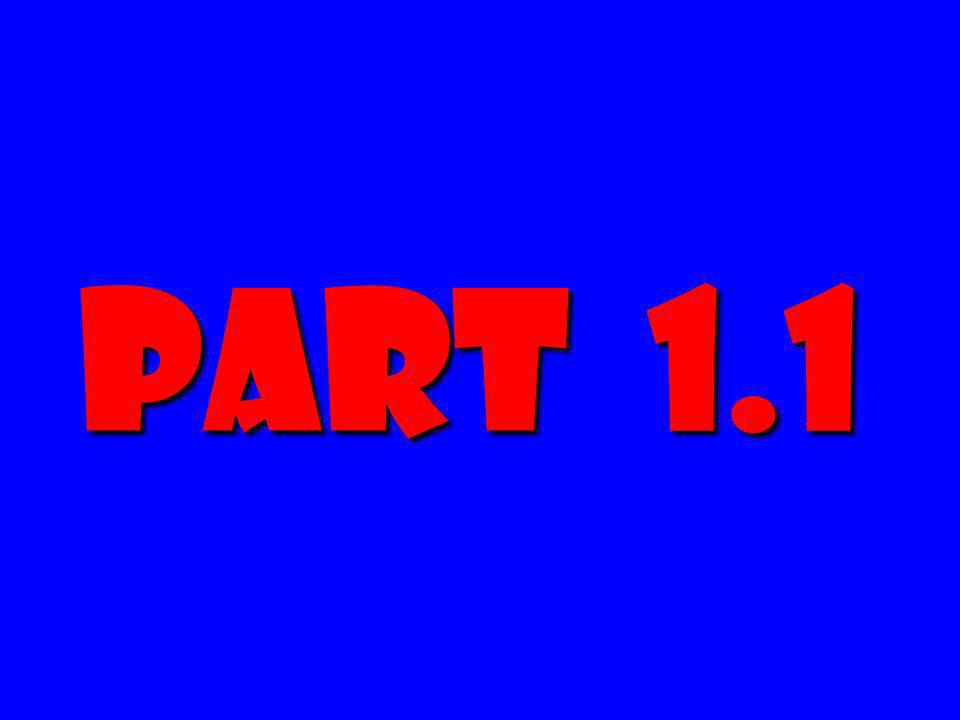The image is a highly simplistic visual likely used for a presentation, characterized by a vibrant and almost glowing bright blue background. Across the center of this backdrop, halfway between the top and bottom, is the bold, blocky text "PART 1.1" presented in a high-impact, cartoonish font. This text is in an intense, bright orangish-red color, further emphasized by a black drop shadow positioned to the right, giving it a textured and somewhat three-dimensional appearance. The design's vibrancy and the sharp color contrast make the image highly noticeable, aligning with its purpose likely as an introduction or transition slide in the presentation.